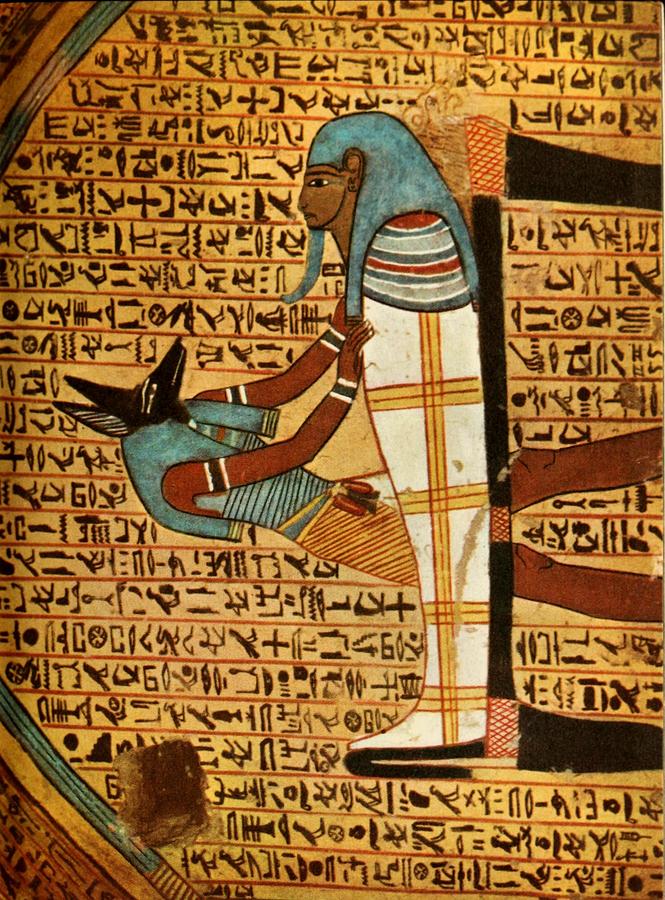The image is a colorful, sideways photograph of Egyptian hieroglyphics painted on the wall of an Egyptian king's tomb monument. Dominating the scene is a sarcophagus standing upright rather than lying flat. To its side, a prominent figure with the head of a black, canine-like creature—most likely Anubis, the Egyptian god of mummification—is placing its hands on the sarcophagus. Anubis, depicted with sharp ears, has a human body with brown-toned skin. The sarcophagus features a figure adorned with a white garment embellished with gold crosses, along with distinctive blue hair and a long blue goatee. Surrounding this central imagery are rows upon rows of intricate hieroglyphic symbols, providing a rich, informative backdrop to the scene.